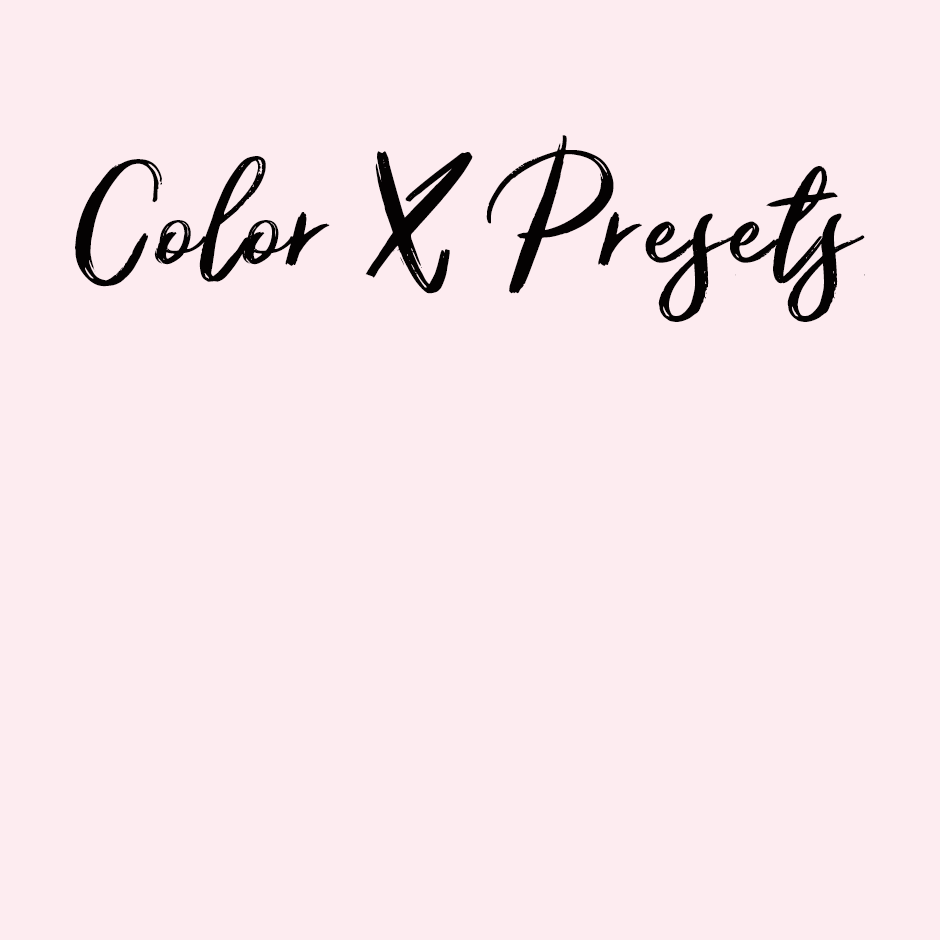The image features a light pink background and is a vertical rectangle close to a square shape. At the top of the image, centered, there is stylized black text with perhaps minor gray and white detailing. The font resembles partial cursive handwriting with paintbrush-like effects, creating small gaps within the letters. The text reads "COLOR X PRESETS," with "COLOR" and "PRESETS" having capitalized initials and "X" being entirely capitalized. The "X" has an extra leg at the bottom and a backward line at the top, adding a modern flair. The letters "S" and "T" in "PRESETS" have distinct features, including larger bottom loops and open tops, with the crossbar of the "T" extending through the opening. The rest of the image remains a blank, open pink space, giving it a clean, minimalist aesthetic possibly designed for social media or clip art purposes.